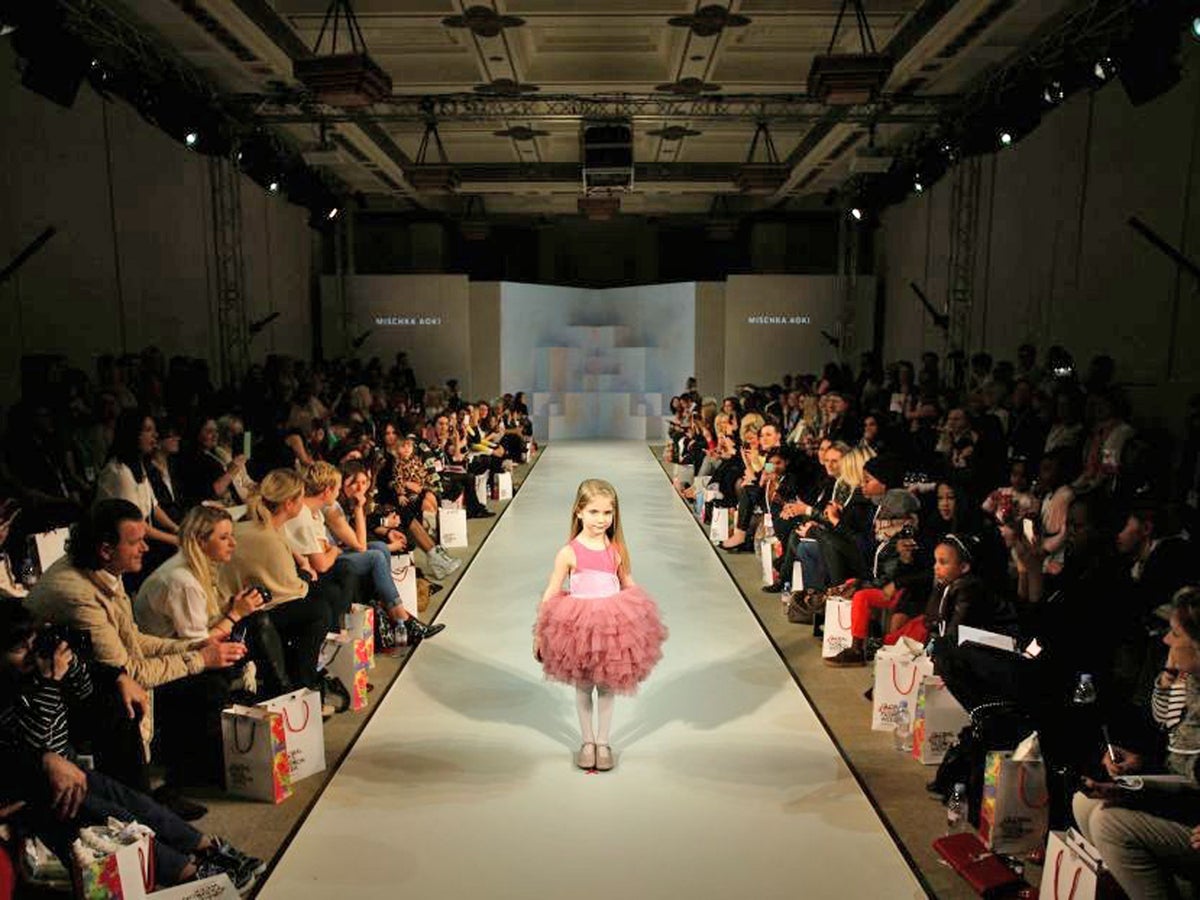In this captivating image, a young girl, approximately five years old with long light brown hair, is confidently strutting down a dazzling white runway, showcasing a striking ballerina-inspired outfit during a bustling fashion show. Her ensemble features a two-tone pink tank top—one shade a darker, richer pink and the other a lighter pastel pink—a frilly, puffy tutu-like skirt, complemented by white stockings and shimmering gold shoes. The room is filled with an attentive audience of at least a hundred people, including both adults and children, many of whom hold white gift bags. Bright strobe lights illuminate the scene, emphasizing the vibrant, colorful attire of the young model. At the far end of the runway, a backdrop with white lettering reveals the name of the designer or the event, though the exact text remains unreadable. The setting exudes the festive, lively atmosphere of a high-energy fashion show dedicated to young aspiring models.